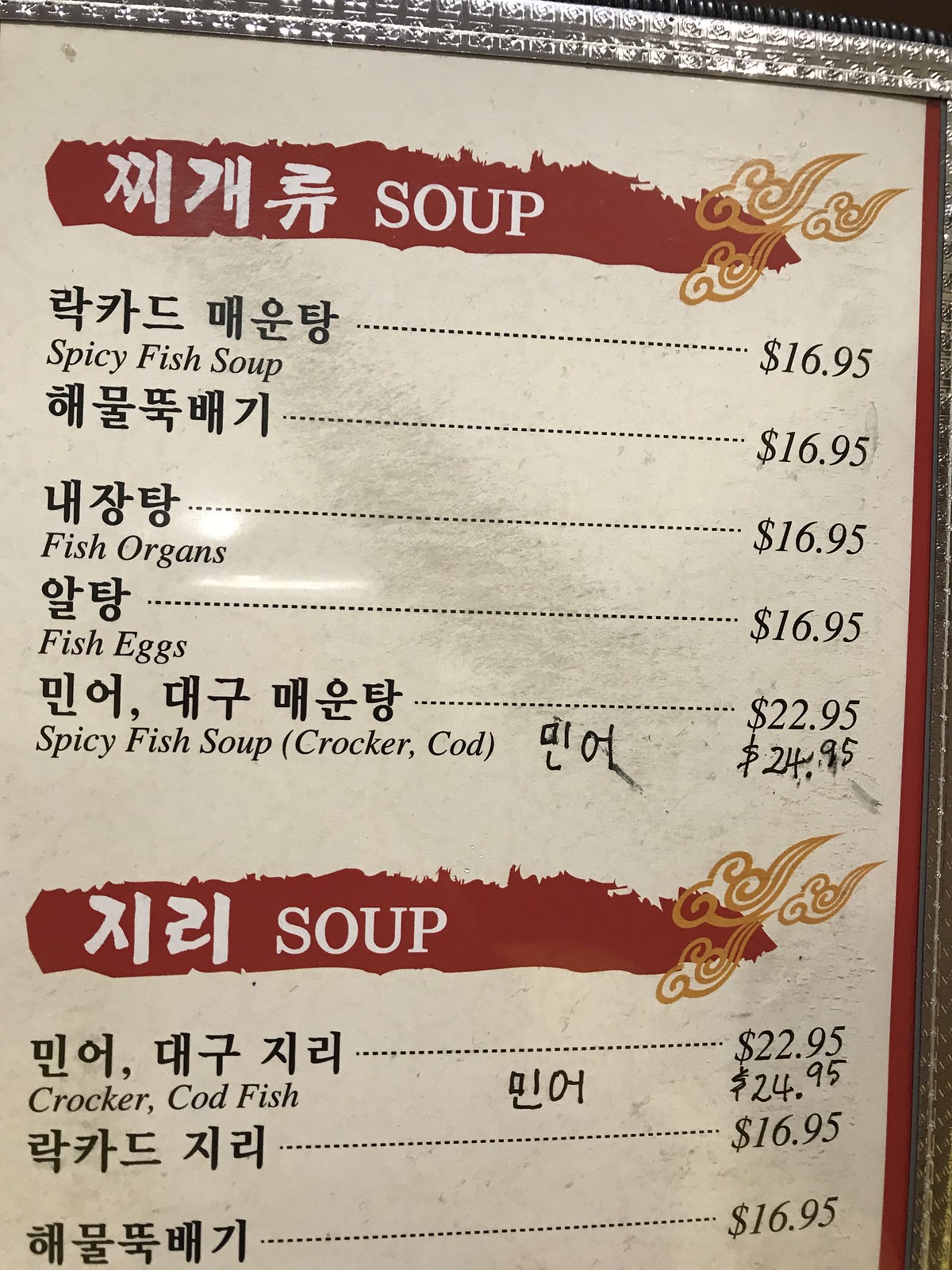The image is a color photograph of a section of a laminated restaurant menu with a beige background and a silver border along the top. A dark red stripe adorns this silver border. The menu features both English and Chinese characters. At the top, in black text, it reads "Soup". Listed below are several menu items with their respective prices:

- Spicy Fish Soup - $16.95
- An unidentified soup (written only in Chinese) - $16.95
- Fish Organs - $16.95
- Fish Eggs - $16.95
- Spicy Fish Soup (Crocker or Cod) - $24.95 (originally printed as $22.95 but overwritten by hand to reflect the updated price)

Further down, another section labeled "Soup" lists:

- Crocker, Codfish Soup - $24.95 (also originally $22.95 but changed by hand to $24.95)
- Two more unidentified soups in Chinese - $16.95 each

The handwritten price adjustments add an element of personalization to the otherwise printed menu.